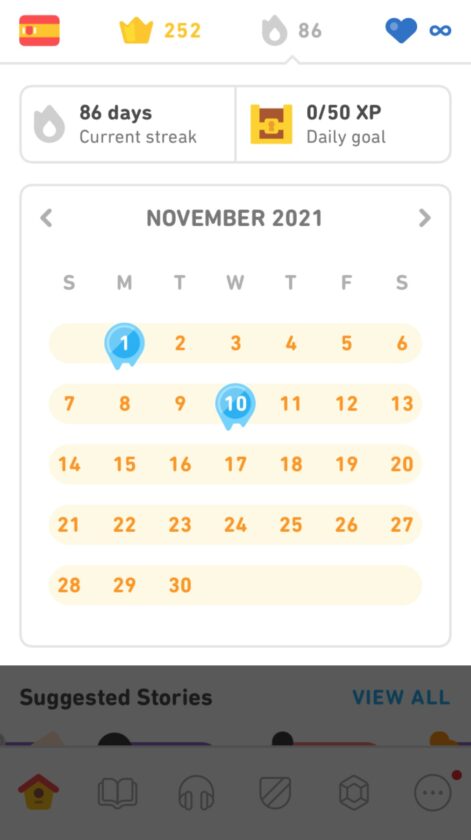This image displays an app interface designed for language learning. At the top of the page, the Spanish flag is prominently featured, with its red and yellow stripes and a crown emblem. Next to the flag, there's an icon displaying the number "252" in gold and gray, likely indicating the total number of units or lessons completed. 

Underneath, the number "86" appears next to a gray flame symbol, signifying the user's current streak of 86 days. A blue heart icon is also present, reinforcing the "86 days current streak" text beside it. Below this, a treasure chest icon notes "0 out of 50 XP," indicating progress towards the daily goal.

The calendar display shows "November 2021" with navigational arrows on either side for switching months. The dates 1 through 30 are listed, and the 1st and 10th are specifically highlighted— the 1st with a blue outline and the 10th with a blue color. All the dates have a yellow line through them, representing the maintained streak.

Below the calendar, there's a section titled "Suggested Stories" with a blue "View All" button. The bottom of the screen features various icons: a home button, an open book, headphones, a badge with a line through it, a multi-sided mirror-like shape, and a circle with three black dots and a red dot, which typically signals a notification.

The image captures both progress tracking and navigation elements of a language learning app, emphasizing user engagement through consistent practice and interactive features.